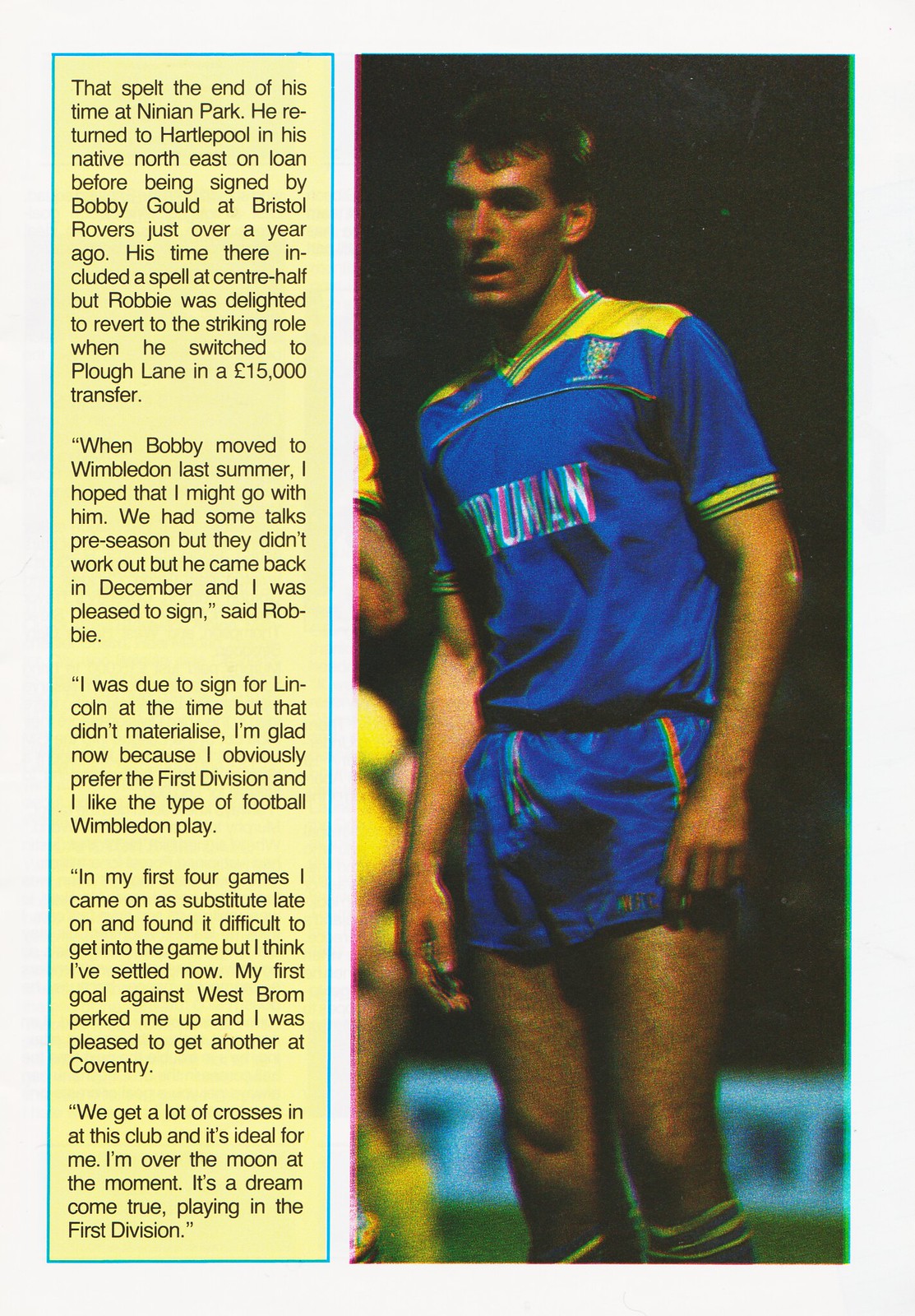This image appears to be a scanned page from a soccer magazine, showcasing a split layout with two distinct sections. On the right side, there is a clear photograph of a soccer player standing on a field, seemingly at rest with his mouth open as if breathing heavily. He has short brown hair and is dressed in a striking blue and yellow jersey with the name "Truman" emblazoned in white letters across the chest, paired with blue shorts and tall socks. Some other players can be seen blurred in the background, indicating an in-game setting. On the left side of the image, there is a lengthy article comprising five paragraphs, written in black letters against a pale cream background and framed by a green border. The text references several football details, including transitions and transfers of players, for instance moving to Hartpool and Bristol Rovers.